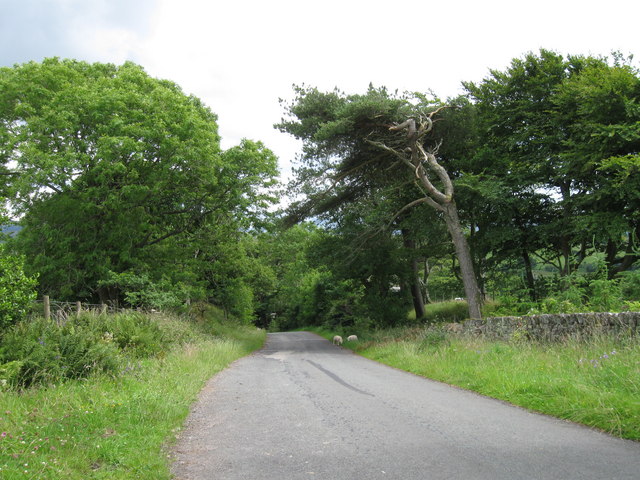The image captures a serene, rural scene featuring a narrow, single-lane country road or long driveway without any line dividers or markings. The road, slightly worn and appearing to be paved some time ago, stretches into the distance, flanked by dense, lush greenery, indicative of spring or early summer. On the left side of the road, a rustic wire fence propped up by brown logs peeks through a thicket of green bushes, accompanied by a strip of green grass. To the right, partially concealed by grass, runs a short stone wall adorned with tall weeds and small purple flowers. In the background, the road is framed by towering trees, their branches thick with green leaves, while a prominent, leafless dead tree stands out, its gnarled branches reaching skyward. The sky above is bright, with patches of blue and fluffy white clouds, indicating a sunny day. Far down the road, a solitary figure can be seen walking towards the camera, and just off to the right, two distant white sheep graze peacefully, lending a rustic charm to the tranquil landscape.